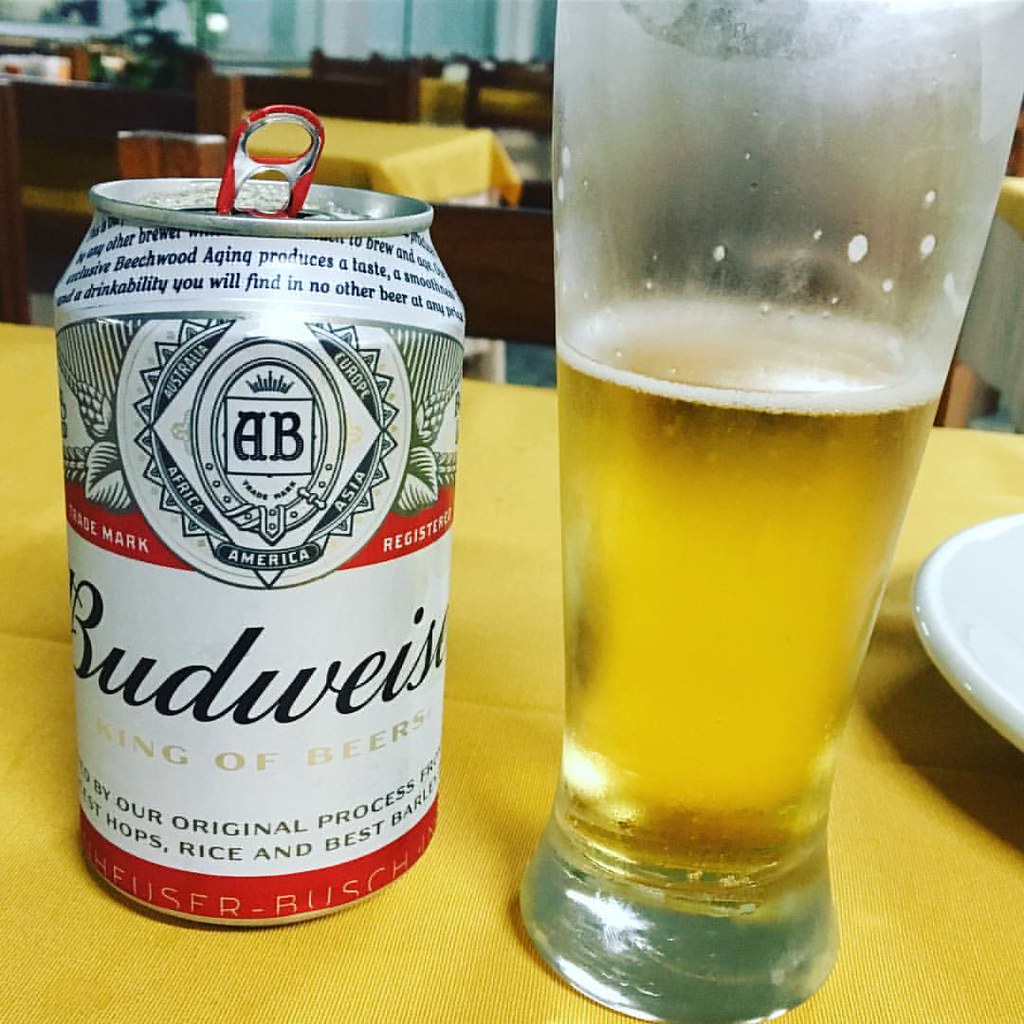This close-up image showcases a Budweiser can of beer prominently positioned on the left side of a yellow tablecloth-covered table. The can displays detailed branding elements including the "Budweiser" logo, the phrase "King of Beers," and portions of its slogan: "Exclusive Beechwood aging produces a taste, a smoothness, and a drinkability you will find in no other beer," alongside "By Our Original Process, Hops, Rice, and Best Barley." The Anheuser-Busch logo crowns the top of the can, with additional branding at the bottom.

To the right of the can, a frosted glass half-filled with beer exhibits noticeable condensation and a white foamy head, suggesting it is freshly poured and chilled. The setup is further detailed by the presence of a partial white plate on the far right edge of the image. The background features a glimpse of additional tables covered in yellow tablecloths with dark wooden chairs pushed in. The setting hints at a larger dining area, with an indistinct, possibly blue and white striped wall adding a subtle backdrop.